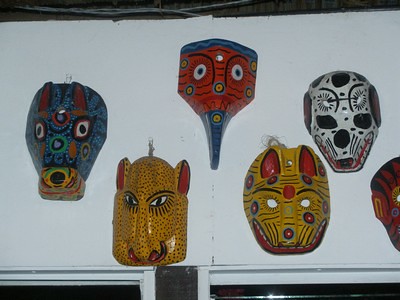This image captures a vibrant wall display of six intricately painted African masks, each depicting a unique and colorful design, prominently hanging on a white wall above door frames. 

Starting from the top left, a blue-hued mask features large white eyes and a red-eared, horse-like nose. Directly below is a vivid yellow mask with black spots, flaunting black eyelashes, a large pink nose, and big yellow ears with pink insides, resembling a stylized cheetah. Next is another yellow mask distinguished by blue and pink circular patterns and adorned with pink ears. Ascending to the center is an orange bird-like face with a long, pointy blue nose and radiant white eyes encircled by sun-like black eyelashes. The top right showcases a black and white mask with skull-like features, evoking the essence of a human skull. Partially visible is a red mask with black striping and human-like eyes.

Each mask's dynamic and abstract patterns enhance the overall aesthetic, highlighting the artistic craftsmanship and cultural significance behind these extraordinary works of art.